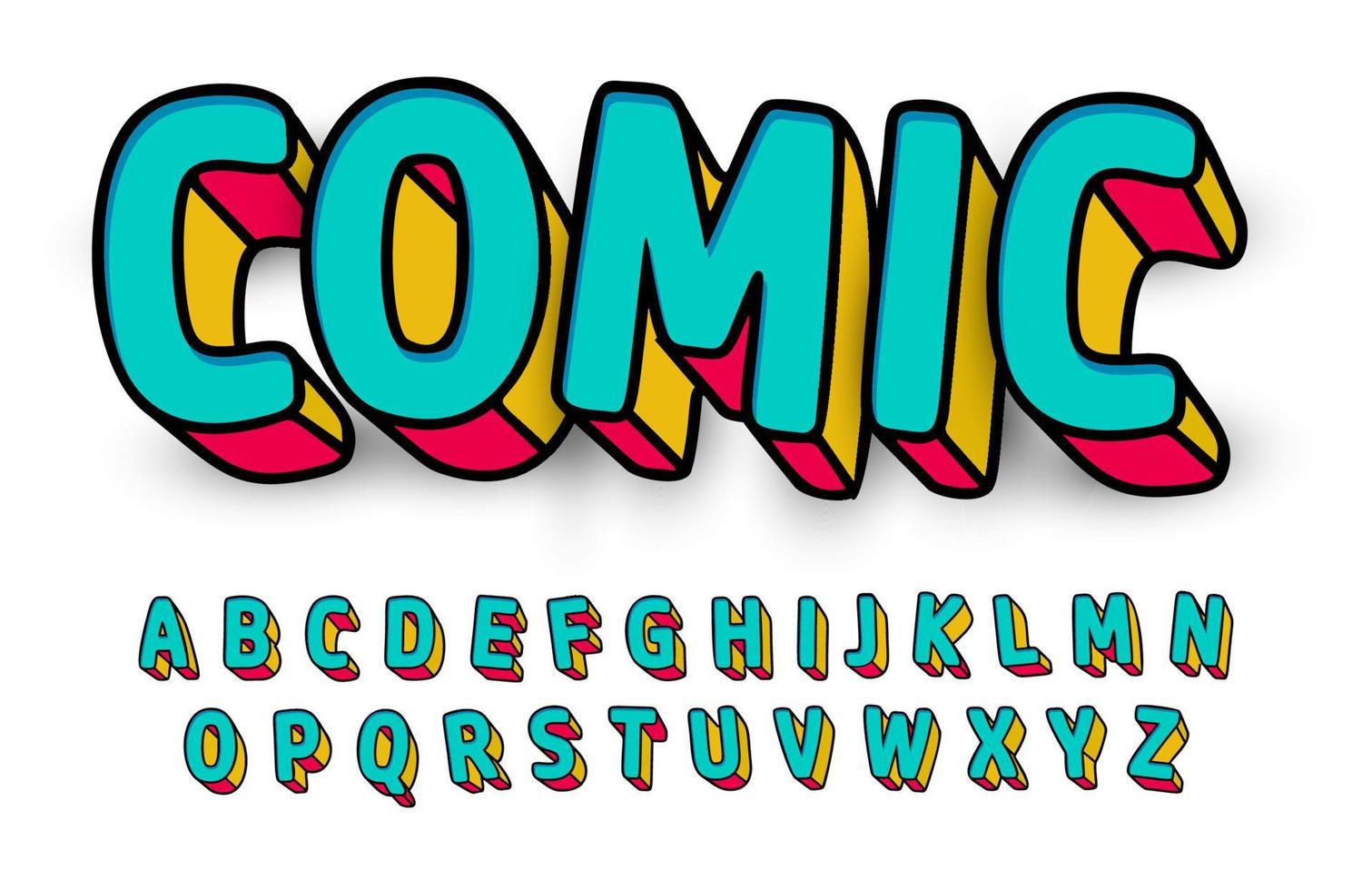The image features a vibrant, cartoonish text against a plain white background. Dominating the top half, the word "COMIC" is prominently displayed in large, bold, capital letters. Each letter of "COMIC" has a primary light blue color with a black outline, and utilizes red on the undersides and yellow on the left sides to create a three-dimensional effect. Below "COMIC," the complete alphabet, from A to Z, is arranged in two rows—A through N on the top row and O through Z on the bottom. The alphabet letters are designed in the same style and color scheme as "COMIC," giving a consistent, colorful, and engaging look. The entire image suggests a playful, educational theme, possibly intended as a learning tool for children to familiarize themselves with the alphabet.